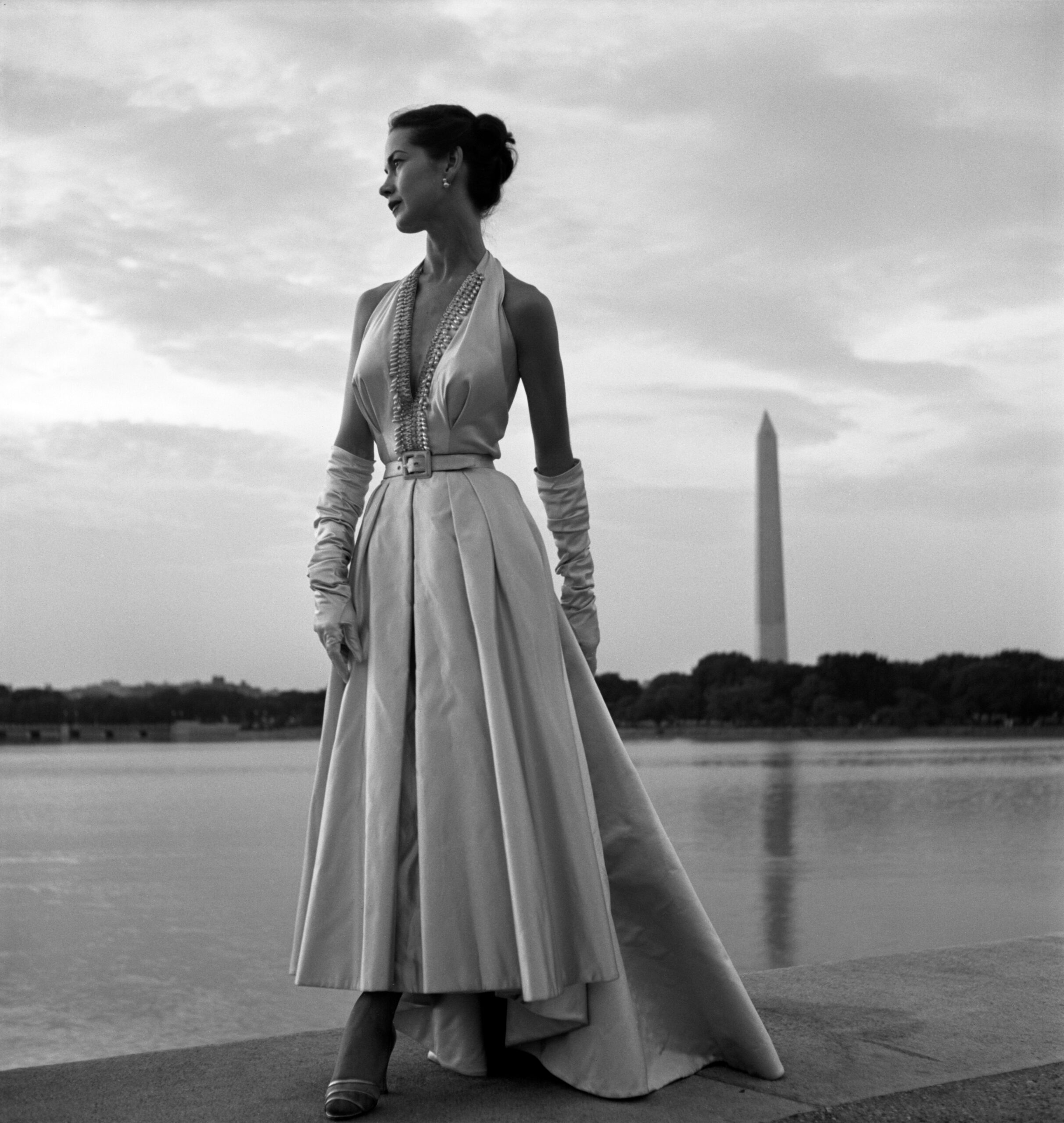In this black and white photograph, an elegant woman stands poised on the edge of a concrete pier near a large body of water, likely the Reflecting Pool, with the Washington Monument visible in the background. She is dressed in a long, sleeveless gown with a voluminous skirt and a V-shaped neckline, cinched at the waist with a belt. Her forearms and shoulders are exposed, and she accessorizes with gloves, high-heeled shoes, and earrings. Her dark hair is styled in a bun at the back of her head. The woman gazes to her right, towards the brightest part of a cloudy sky streaked with clouds. Her stance, with one foot slightly forward and visible from under her dress, and the sophisticated attire, suggests she is either posing or in deep contemplation.